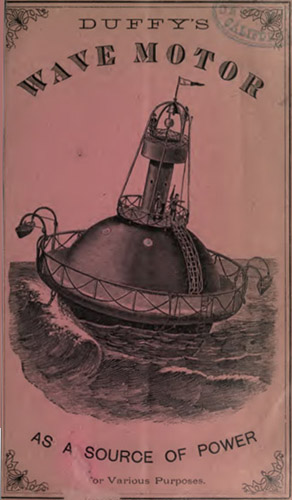The image depicts an antique piece of ephemera with a pale, grayish-rose background. At the top, bold black capital letters spell out "DUFFY'S," followed by larger, curved letters that say "WAVE MOTOR." The corners of the paper feature intricate black filigree designs. Below the text, an illustration likely rendered in gray tones, resembling a lithograph or etching, shows Duffy's Wave Motor, a buoy-like contraption with a bulbous base and a pointed top featuring a small flag. The motor appears to be large enough to accommodate two men and is set against a backdrop of rocking ocean waves. Directly below the illustration, text reads "AS A SOURCE OF POWER." There is a discernible ink stamp in the upper right corner, potentially indicating "California." The overall color of the paper suggests it has aged to a pale, pinkish-purple hue, though the image might have been originally more yellowed. This imagery serves as an advertisement for the innovative Duffy's Wave Motor, highlighting its potential as a unique source of power.